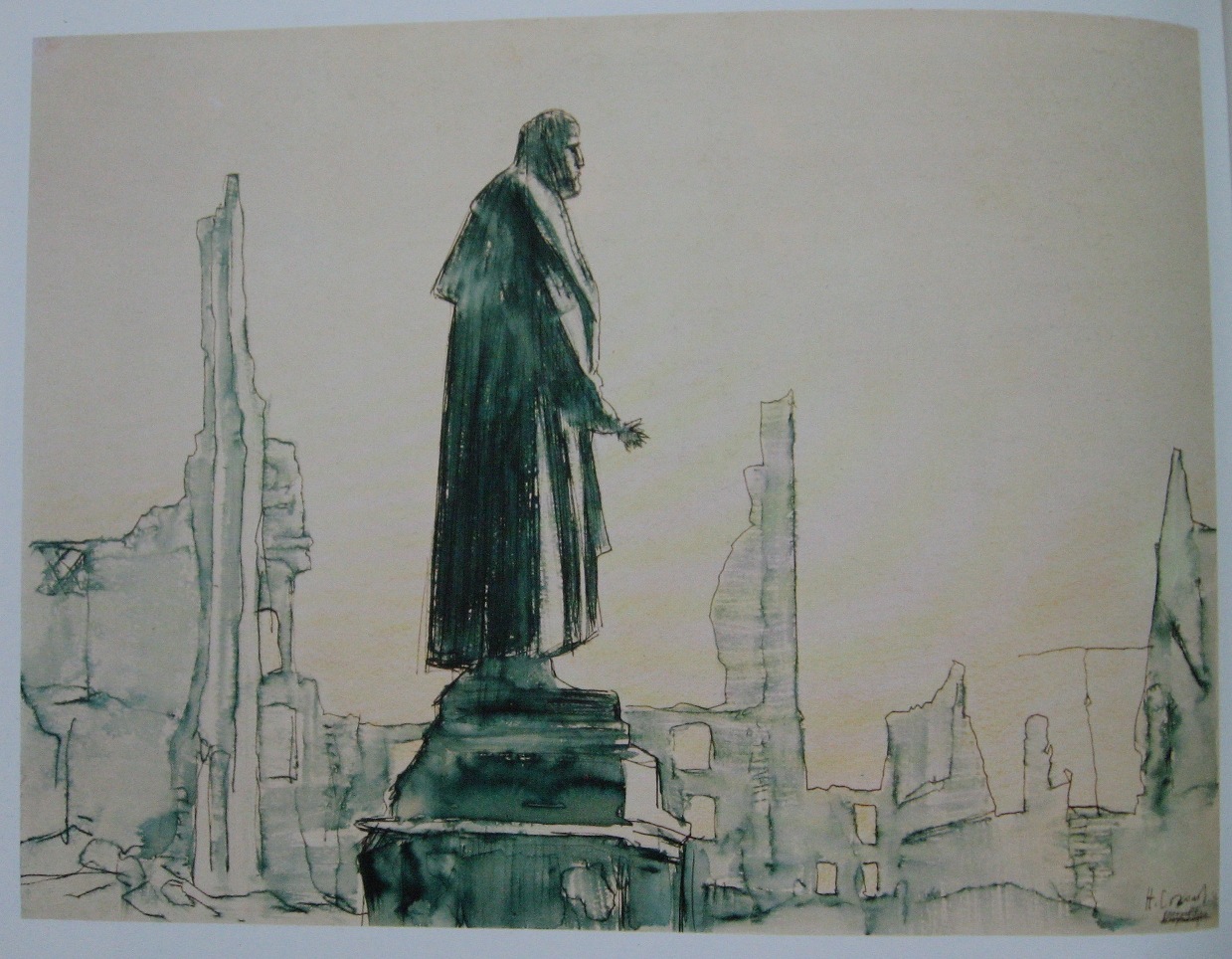This is a detailed drawing or watercolor artwork on a large, beige or light brown sheet of paper. The background of the artwork is a bluish-gray color. At the center of the composition is a statue of a male figure, standing on a square pedestal that appears to be made of stone, rendered in shades of gray and black. The statue is shown in profile, facing right. The figure is dressed in a long robe or gown that flows around him, with chin-length straight hair, suggesting a classical or ancient motif. His hand is slightly extended forward, perhaps in a gesture of greeting or beckoning.

In the background, there are outlines of abstractly drawn buildings with minimal detail, resembling old ruins or modern skyscrapers, characterized by their crooked lines and simple, child-like rendering. The buildings are depicted with tall vertical forms and basic window outlines, contributing to a sense of depth and timelessness. The overall monochromatic palette, using shades of gray and black, ties the composition together, giving it a cohesive, almost dreamlike quality.